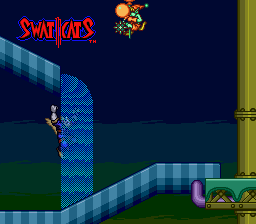The image is a screenshot of a computer game featuring vibrant colors and intricate details. Dominating the upper left-hand corner, there is a logo with red letters outlined in blue that reads "SWAT CATS," with a "TM" symbol beneath it and three lines separating the words "SWAT" and "CATS." The background of the logo is situated within a purple rectangle. Along the right edge of the image, a tall, vertical, light green cylinder extends from top to bottom. This cylinder, or pipe, connects to a network of variously colored pipes: a blue-striped pipe with water running from it on the left, and a purple pipe linked to an olive-colored pipe in the center. The game's background includes a blue frame or wall with streaks of light and dark blue, traversing from the left side, turning right, and engulfing a character who is blue, brown, and red-gray in color. An orange-green figure blowing a bubble is present in mid-air, adding a playful element to the scene. The overall scene is dynamic and colorful, integrating elements of green clouds and brown and green logs, evoking a whimsical game environment.